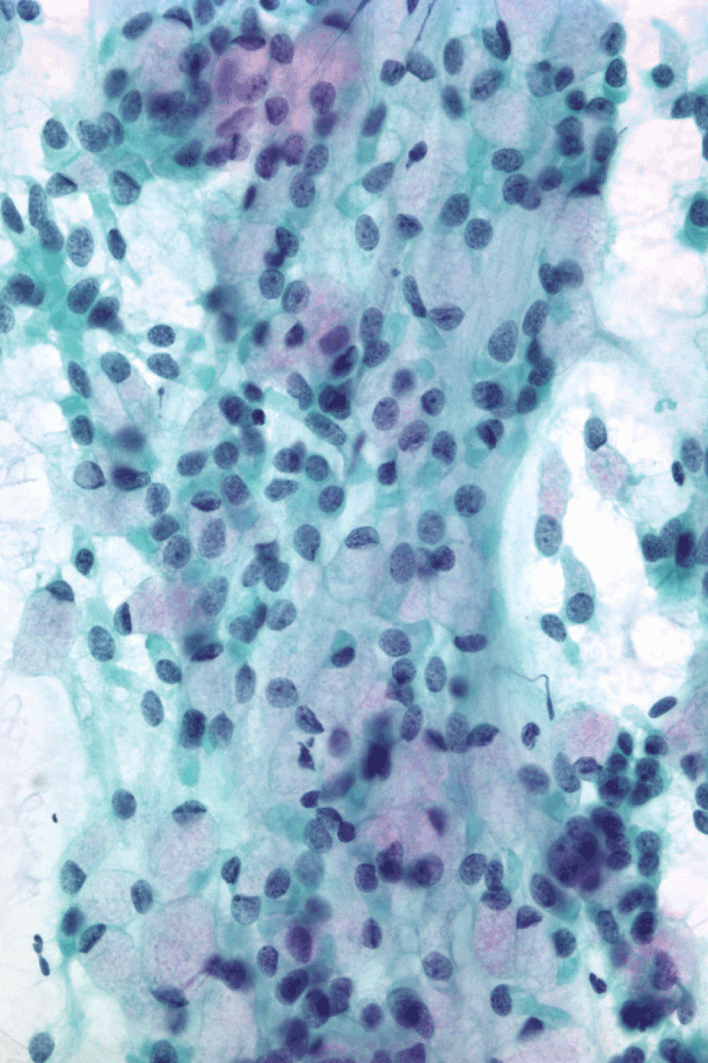This abstract painting presents a symphony of colors and forms on a predominantly white background, creating a scene that resembles both nature and microscopic cellular structures. Dominated by shades of aqua, teal, and dark green, the composition features a prominent green stalk that rises from the bottom to the left, adorned with smaller branches. Interspersed throughout this organic form are black oval spots, reminiscent of fingerprints, lending a textured contrast.

The painting also incorporates various green tones, from light seafoam to deeper hues, along with dark blue and gray splotches that add depth and complexity. Scattered across the canvas are indistinct blobs of purplish-rose and red, which appear along the middle and near the bottom right, blending seamlessly into the green backdrop. These reddish elements, along with a pair of faint red orbs near the top left, add a subtle glow to the piece.

The artwork's overall abstract nature evokes imagery of both stained glass and biological cells, creating an enigmatic visual experience that captures the imagination with its intricate and vivid interplay of colors and shapes.